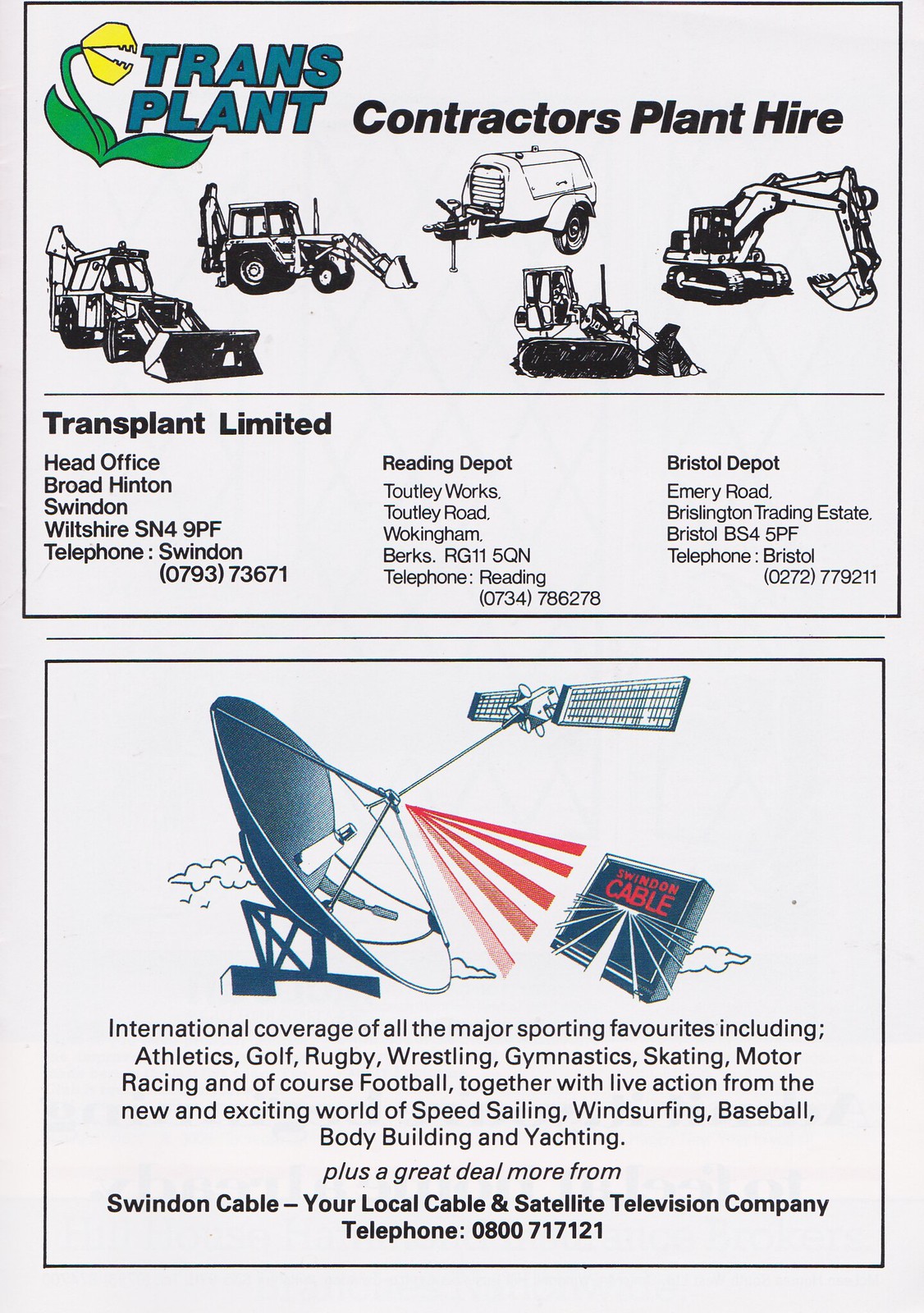This image appears to be a page from a magazine or a flyer, featuring two distinct advertisements bordered in black. The top section promotes Transplant Limited, a contractor's plant hire company. The advertisement has a grayish background with the company name "Transplant" prominently displayed in blue and black outline. Accompanying the name is a logo resembling a Venus flytrap with green leaves and a yellow flower, which also suggests the scoop of a large bucket loader. The ad lists various construction equipment rentals available, such as tractors and bucket loaders. It also provides the company’s head office address in Broad, Hinton, Swinton, Wilshire, SNF49PF, and the contact number, Swinton D793-73671. Additional depots are mentioned, including Reading and Bristol, with respective addresses and phone numbers.

Below the Transplant ad is a separate section devoted to Swindon Cable, a local cable and satellite television provider. This part of the advertisement features a large, conspicuous satellite dish and red lines indicating signal transmission. It touts international coverage of all major sporting events, such as athletics, golf, rugby, wrestling, gymnastics, motor racing, football, speed sailing, windsurfing, baseball, bodybuilding, and yachting. Contact information for Swindon Cable is also provided, including the telephone number 0800-717-121.

The overall color scheme of the flyer includes shades of gray, blue, yellow, green, tan, and black, and the entire page is visually dense, giving it the appearance of a comprehensive advertisement spread.